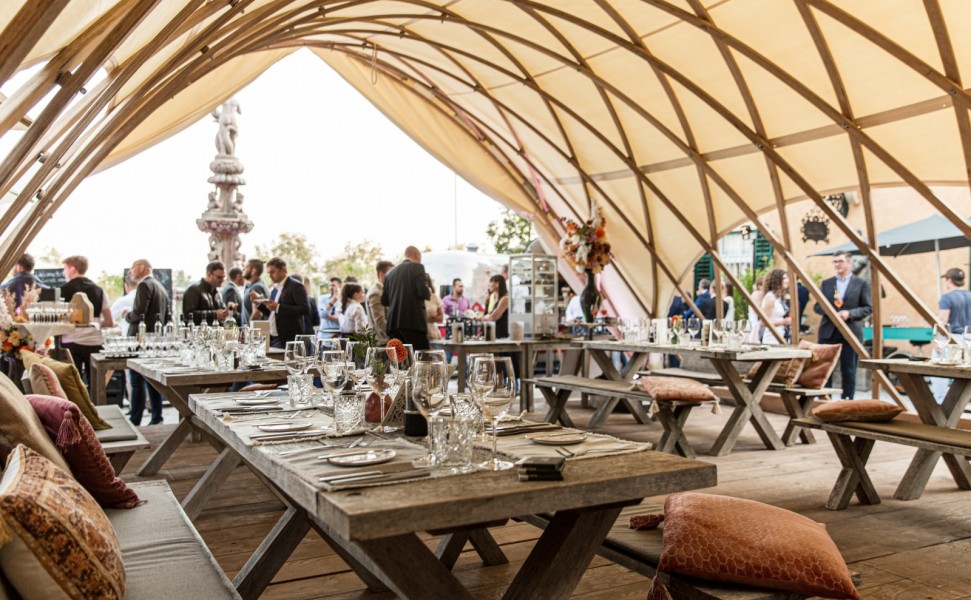The image depicts an outdoor scene featuring a large wooden gazebo with a cream-colored tarp covering its lattice frame, which extends from the ground upward and then back down. Inside the gazebo, there are approximately five picnic tables adorned with decorative pillows on the benches and set with wine glasses, dinnerware, and silverware, indicating a meal is about to take place. The setting appears to be for a formal event, possibly a wedding reception or a party, as evidenced by the guests dressed in formal attire, including suits, slacks, and dresses. In the background, a two-tier marble fountain with a statue of a person atop is visible, adding an elegant touch to the picturesque, sunny yet hazy day. The shadows are soft, enhancing the serene and festive atmosphere of the gathering.